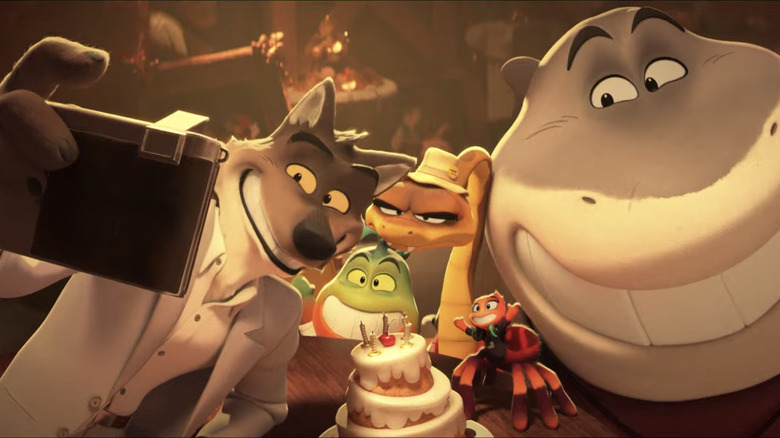The image depicts a vibrant scene from a 3D animated cartoon with a poster-like quality. At the center of the scene is a wooden table with a multi-tiered birthday cake, surrounded by a colorful cast of anthropomorphic characters. On the left, a cheerful wolf wearing a cream-colored sport coat and an open shirt is capturing a selfie with a camera or phone. This wolf has a big smile, pointy ears, and white cheeks. Next to him is a large gray hippopotamus-like character with a massive head and a broad toothy grin. Further along, a yellow snake sporting a cap and squinty eyes can be seen, showing off its fangs. There's also a quirky green character with large jaws and greenish eyes peering from behind. In front of the cake, a small red crab-like creature with black accents and a tiny orange head sits on the table. The background hints at more tables, suggesting the setting could be a restaurant or a bar. Overall, the image is beautifully detailed, showcasing the characters celebrating a birthday party with vibrant, brilliant colors.